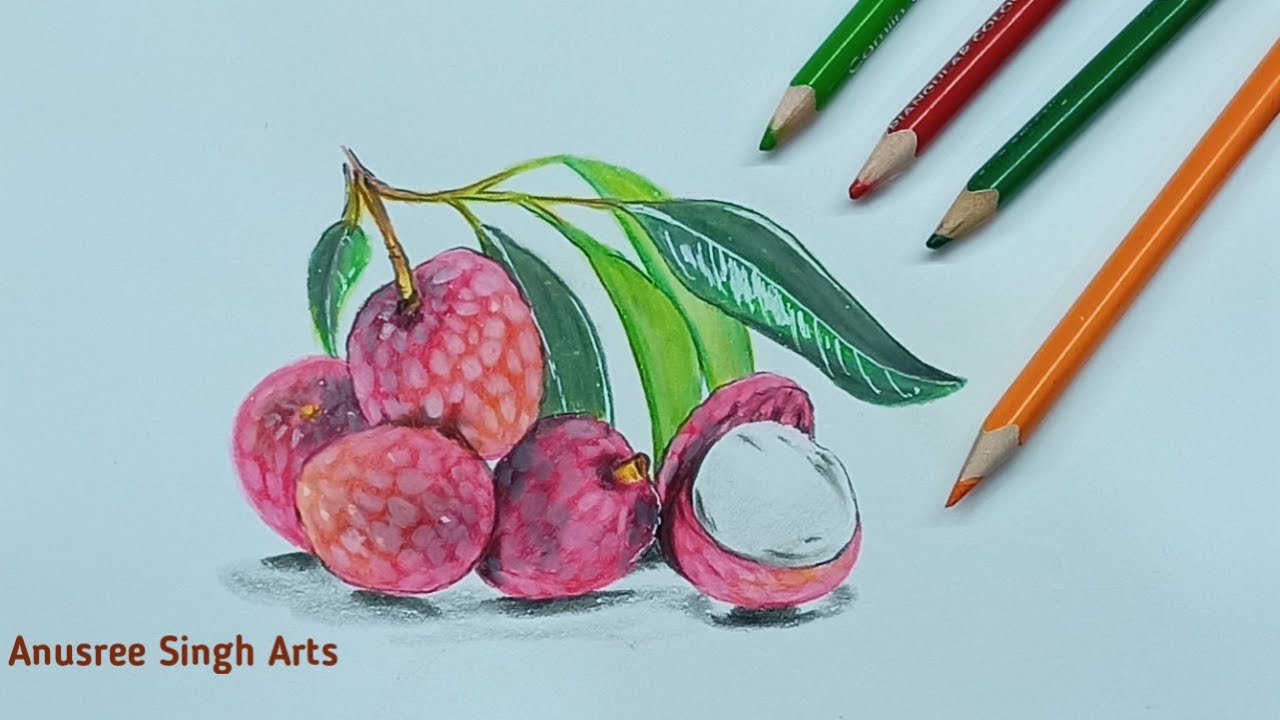This image captures a detailed colored pencil drawing, signed in the bottom left corner with the name "Anusree Singh Arts" in a reddish-brown font. The artwork features five reddish fruits, possibly raspberries or strawberries, each with green leaves and stems. One of the fruits is cut open, revealing a white seed inside. The fruits are either stacked or arranged together with intricate shading and coloring. Along the top right corner, four colored pencils—light green, red, dark green, and orange—are shown, indicating they were likely used to create the artwork. The orange pencil appears the least used, as it is sharper compared to the duller tips of the other pencils. The background of the image is a solid gray, enhancing the vividness of the fruit and pencils.